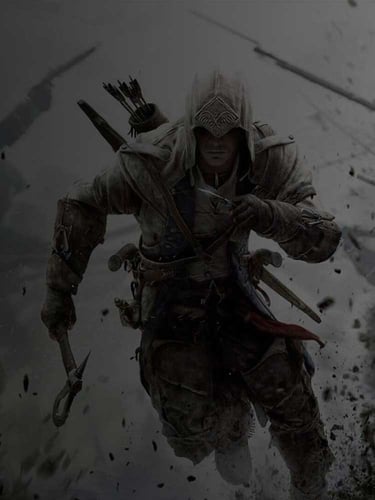The image is a close-up screenshot from a grayscale video game or cartoon, depicting a light-blonde, Caucasian warrior mid-run in a war-torn setting. The background is shrouded in dark, gray rubble, evoking a grim atmosphere of chaos and conflict. The warrior is clad in a dark, uniform-like outfit featuring a hood that partially covers his eyes; the hood is marked with a distinct diamond-shaped symbol at its tip.

In his right hand, the warrior wields a tomahawk-like axe, while his left hand gripes an instrument resembling a blade or needle. Strapped to his back is a bow and quiver filled with arrows. Along his waist, two guns are holstered on either side, contributing to his heavily armed appearance. His gear also includes a sword at his waistline. Additionally, a piece of cloth with a hint of red hangs from his attire, standing out as the only colored element in the predominantly gray-scale image. The overall composition suggests the warrior is escaping or charging through the chaotic battleground.